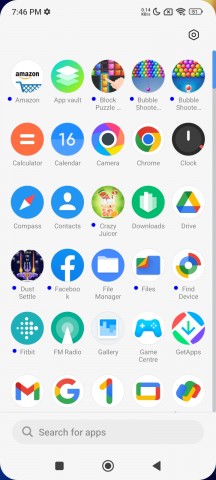This screenshot from a smartphone features a light gray background. In the upper-left corner, a gray font displays the time as 7:46 PM. On the right side, a battery icon shows a 51% charge, alongside the Wi-Fi signal icon, a crescent moon indicating Do Not Disturb mode, and an unidentified icon resembling a square with a slanted upper-right corner.

The screen showcases the user's apps, organized in a 5-column by 6-row grid, creating a vibrant mosaic of app icons. In the top-left corner, the Amazon shopping app icon is visible, adjacent to a green circle labeled "App Vault." Notably, the third row includes a blue circular icon for the Compass app, and another blue background icon for Contacts. The familiar blue Facebook app icon with a white letter "F" is also present.

At the bottom of the screen, various Google apps are displayed: Gmail, the main Google app, Google One, Google Chrome, and another unidentified app featuring Google's signature colors—green, blue, yellow, and red. Below these is a light gray, rounded search box that reads "Search for apps" in gray font, accompanied by a search icon, characterized by a small magnifying glass.

Overall, the shot captures a well-organized, colorful array of frequently used applications on a personal smartphone interface.